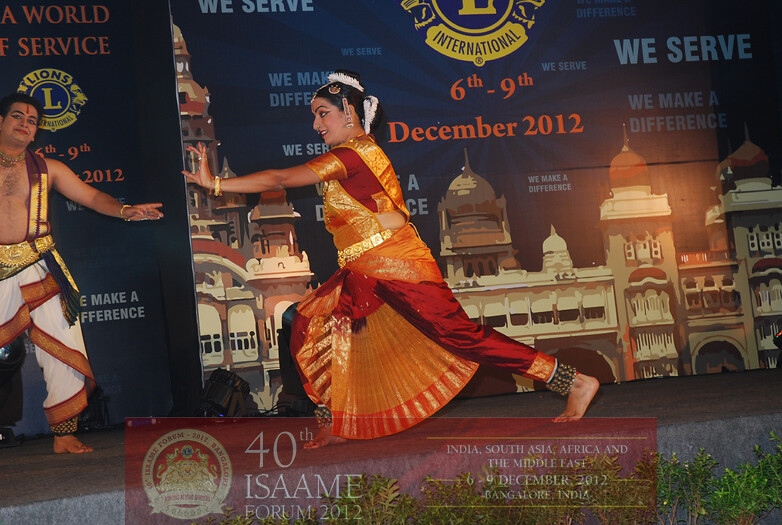"This color photograph, in landscape orientation, vividly captures two people dancing on a stage, emphasizing representational realism. The central figure is a woman in her 30s or 40s, facing left and lunging forward with her left arm raised. She is barefoot and adorned in an ethnic costume featuring a gold skirt over red satin pants. The man on the left side of the image complements her attire with an ethnic costume that includes a gold vest over an open chest and white pants with a red band at the bottom. The background showcases event banners with elements such as the Lions Club logo, dates 6-9 December 2012, and phrases like 'WE SERVE,' along with Indian architectural motifs. The bottom of the image displays a red banner with white foreign-language text, ‘40th ESAAME Forum 2012,’ and mentions regions including India, South Asia, Africa, and the Middle East. The event took place in Bangalore, India, adding cultural and temporal context to the dancers' traditional performance."